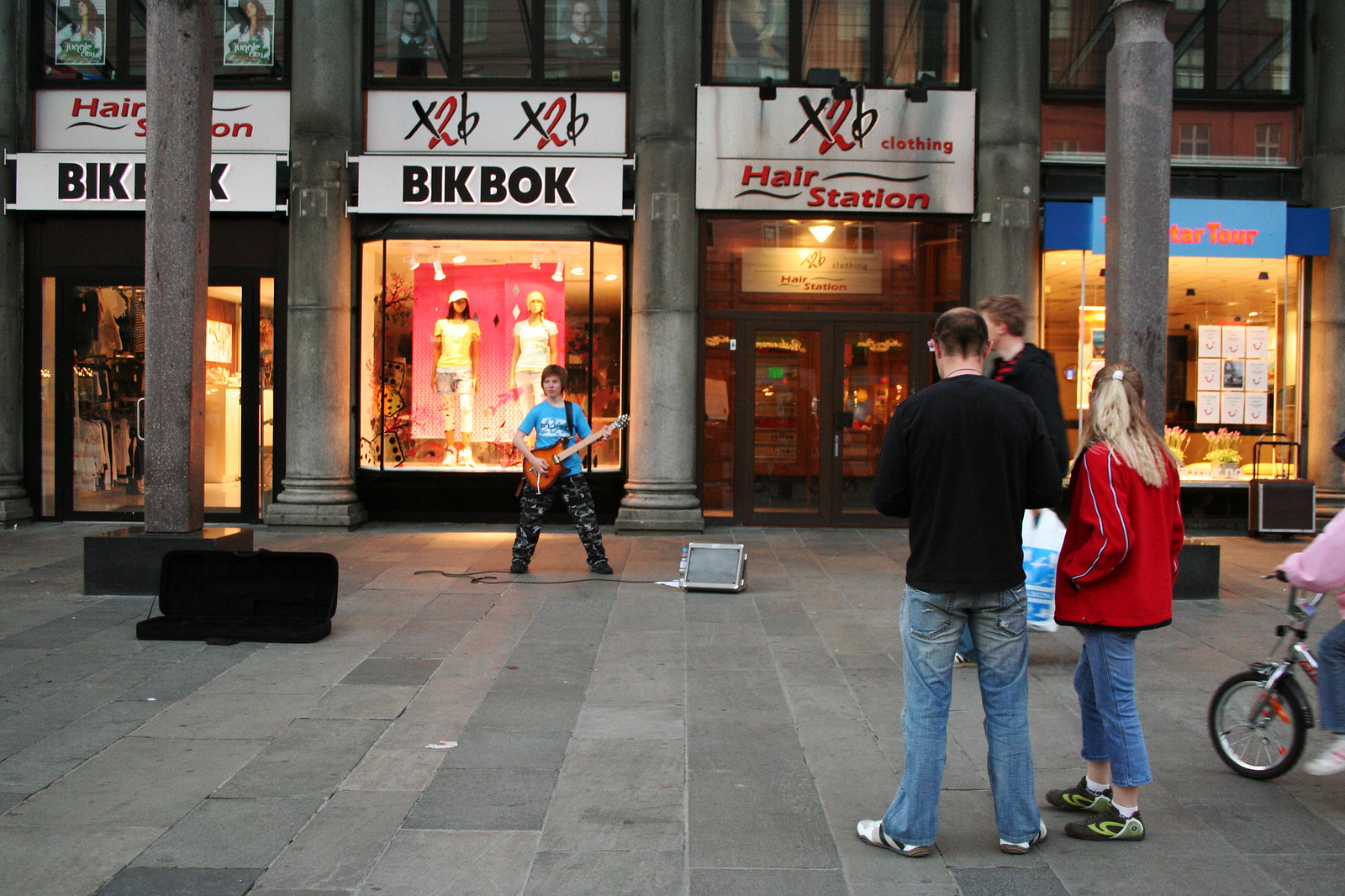In this detailed full-color photograph, taken outdoors in a bustling city plaza or mall at dusk, a young boy is seen standing at the front playing a bass guitar, likely a Gibson, which is brown. He is dressed in a blue t-shirt and black and white pants, with a small amplifier positioned beside him, suggesting he is performing to earn some money. Surrounding him are five onlookers; to the right, a girl with blonde hair and blue jeans is wearing a red jacket, while directly beside her is a man in blue jeans and a black sweatshirt. Another man, also in dark clothing, is observing the scene, and a child is seen on a bicycle, adding to the lively atmosphere.

The backdrop consists of a series of storefronts with distinct signage. There are inscriptions such as "Star Tour" written in red on a blue background and "X2B", along with names like "Bicboc" and a "Hair Station," indicating a mix of different commercial outlets including clothing stores and a hair salon. Inside one of these stores, two female mannequins are spotlighted, further enhancing the vibrant commercial setting of the photo. The cloudy sky above suggests it might be twilight, adding a dynamic and somewhat serene feel to the scene.